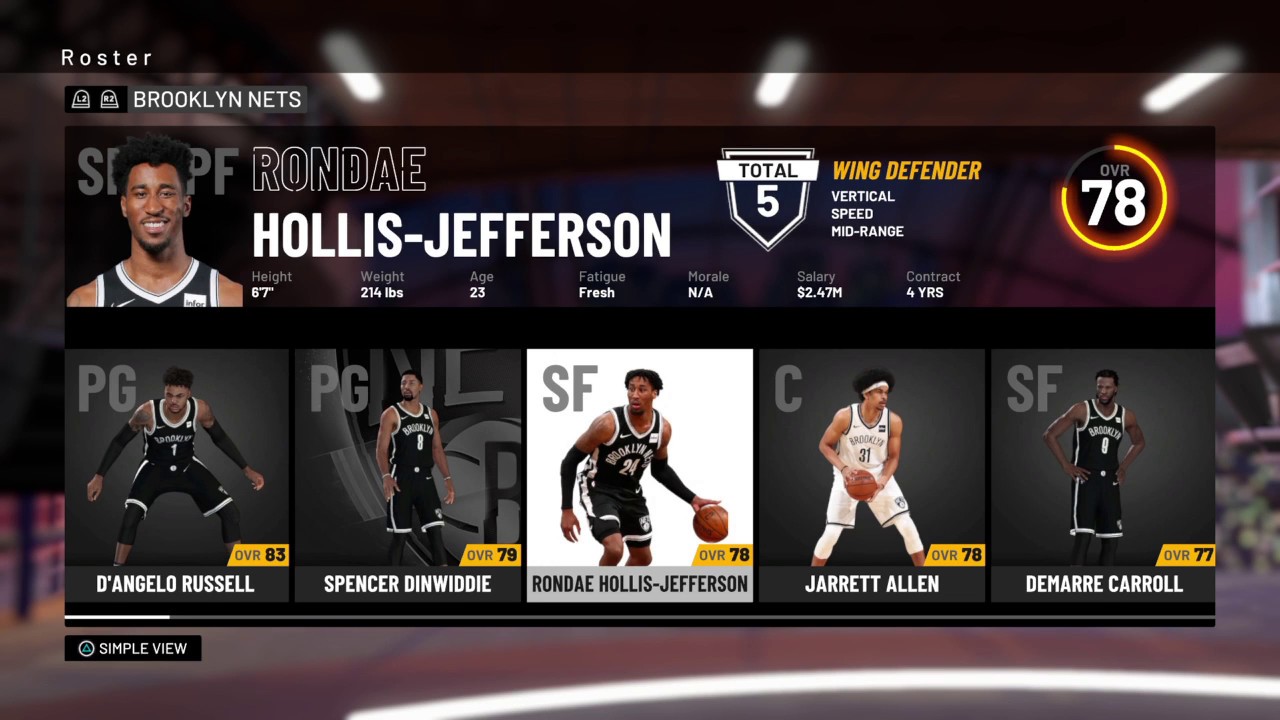**Detailed Descriptive Caption:**

This is a highly detailed screenshot from a sports video game featuring the Brooklyn Nets team. The focus is on player Ronde Hollis-Jefferson. The player’s profile is prominently displayed at the top of the screen. On the left side, there's a picture of Ronde Hollis-Jefferson, and next to it, his name is clearly written. Below his name, a list of his key stats is provided: his height is 6'7", he weighs 214 pounds, his age is 23, his fatigue status is marked as 'fresh', his morale is labeled as 'NA', his salary is $2.47 million, and his contract length is four years.

Adjacent to these statistics is a shield icon with the text "Total 5" on it. Next to the shield icon, the words "Wing Defender" are highlighted in orange text. Below this, in white text, there are the words "Vertical", "Speed", and "Mid-Range". On the far right of the screen, a circular bubble is shown with the number 78 in white text. The outline of this circle is predominantly neon orange, covering about three-fourths of its circumference.

Below Ronde Hollis-Jefferson’s details, there is a second banner showcasing five other player profiles with their corresponding pictures. From left to right, the players are D'Angelo Russell, Spencer Dinwiddie, Ronde Hollis-Jefferson (repeated from the first banner), Jarrett Allen, and DeMarre Carroll.